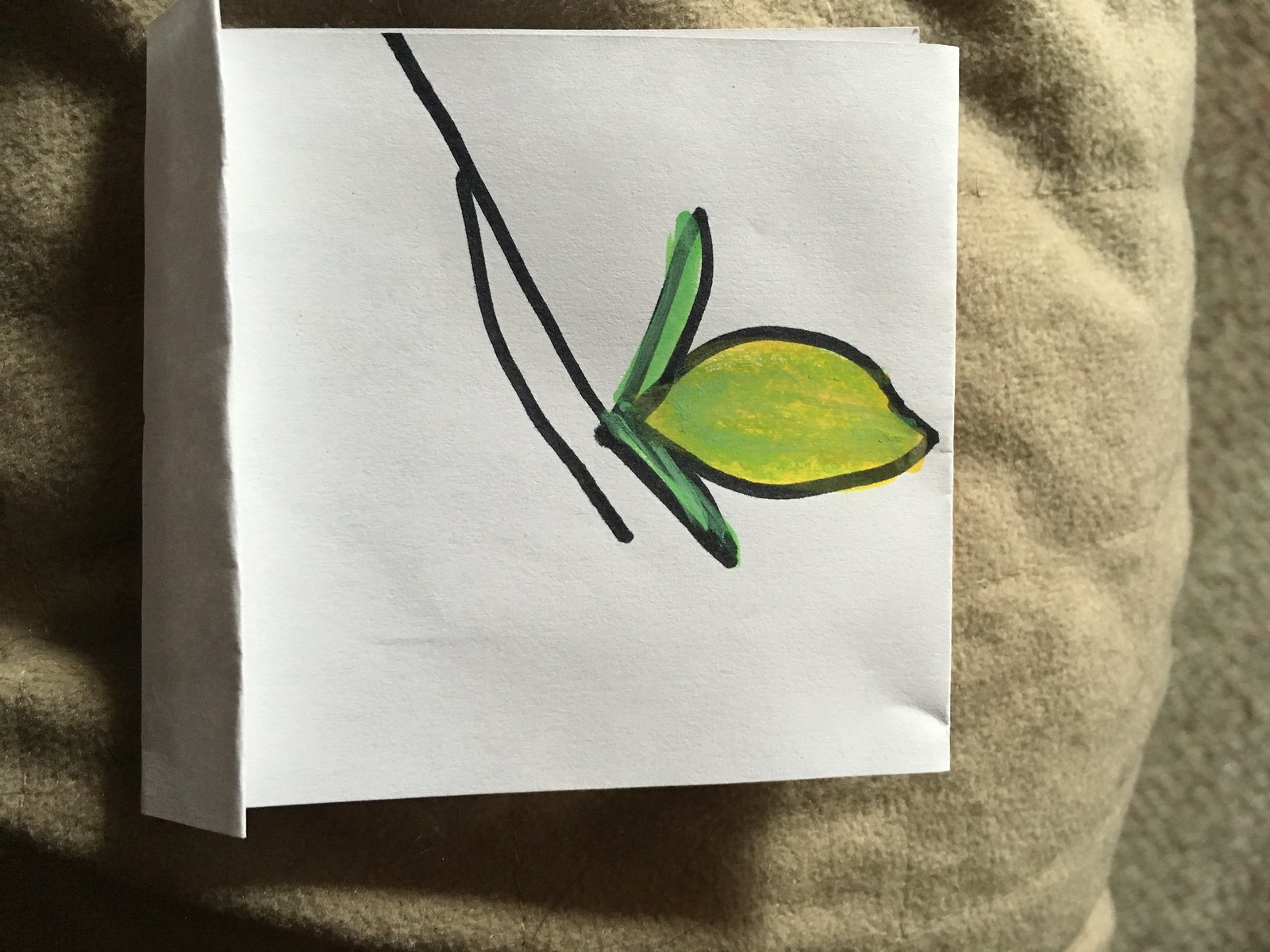The photograph depicts a hand-drawn image on a folded piece of white paper, resting on a beige cloth surface, likely a blanket, with a hint of earth-toned carpeting visible beneath. The paper has been folded multiple times, suggesting it was originally a long, narrow sheet now turned into a square, with an additional fold at the bottom. The artwork on the paper features a black stem extending from the top of the page, culminating in a yellow flower with two green leaves. The outlines of the flower and leaves are meticulously drawn in black marker, while their interiors appear to be colored with a combination of marker and possibly paint, giving them a mixed-media feel.